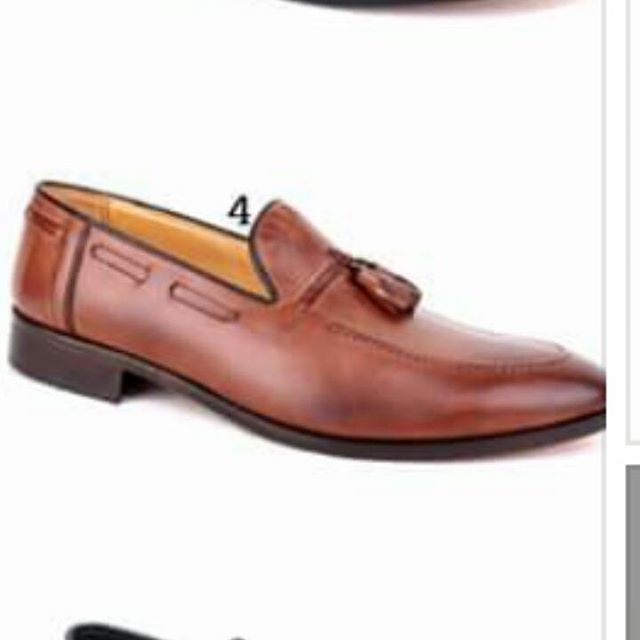This image appears to be a scanned, somewhat blurry and low-resolution photograph that suggests it might originate from a catalog or magazine, likely promoting shoes. The focus is on a brown slip-on loafer centrally positioned with its toe directed to the right and heel to the left. The shoe is crafted from rust brown leather without laces, featuring a darker brown sole. The inside of the shoe contrasts with a lighter tan or cream color. A prominent black number "4" is located just above where the tongue of the shoe meets the opening. The background of the image is predominantly white, with hints of additional items: a curved shadow in the narrow upper right strip and a black heel loop of another shoe in the bottom left. The toe of the featured shoe is slightly cut off by a thin vertical grey line, which aligns with magazine-style sectional dividers, and a thicker grey band appears in the bottom right portion of the image.